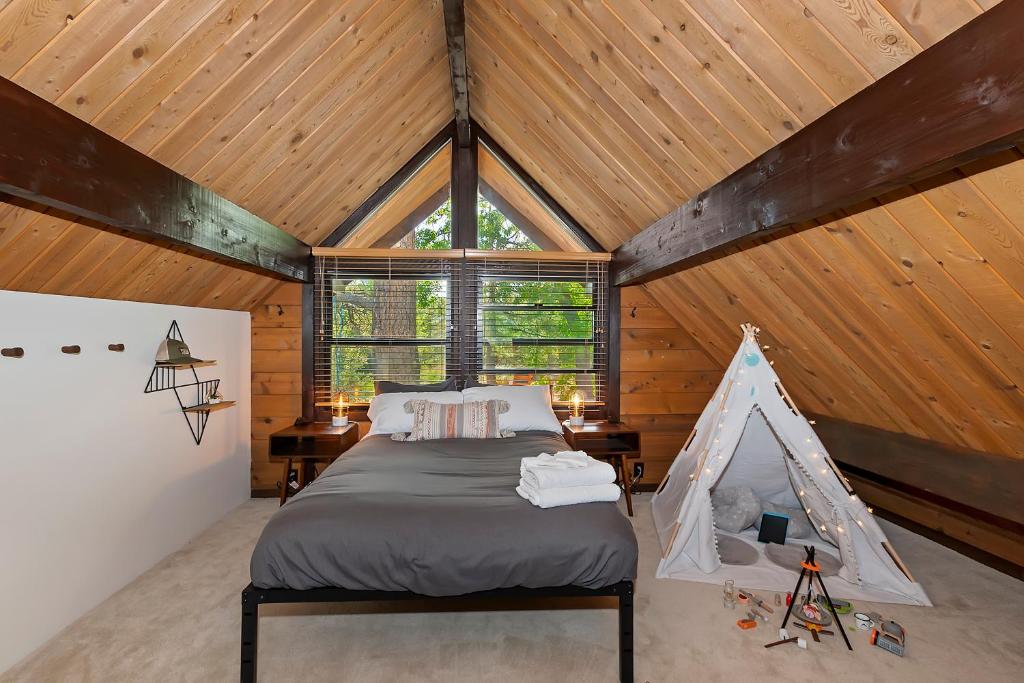This is a detailed photo of an attic bedroom with a rustic, homely feel. The room features an A-shaped ceiling with a dark brown beam at the peak, flanked by light brown wood frames extending up the sides. The beige carpet grounds the room, where the focal point is a black metal-framed bed, adorned with a gray comforter, two white pillows, and a throw pillow with vertical muted stripes. Situated at the foot of the bed are neatly placed white towels.

To the right of the bed, a white teepee tent, adorned with twinkle lights and gray pillows inside, creates a cozy nook, possibly for children. Adjacent to the tent is a charming miniature campfire setup complete with pretend fire, flashlight, and a little mug. On the left side wall, which is completely white, a couple of triangle shelves hold a hat and some hangers. Opposite, on the right side of the room, there are two windows flanked by blinds, offering a view of lush green trees outside.

This picturesque attic room exudes comfort and adventure, blending simplicity with playful elements for a delightful retreat.